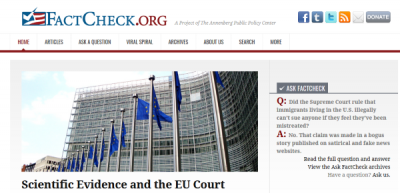The image features an American flag with a checkmark superimposed on it, positioned next to the text "FactCheck" in blue, followed by ".org" in red. Adjacent to this, there are some small, unreadable gray words. On the right side, various logos are displayed: the Facebook logo, an icon with a "T," a lighter blue square containing a darker blue element, an orange logo with a dot and two curved lines, and an almost invisible envelope outlined in light gray. Below these, there is a gray rectangle containing illegible text. Across the top of the image are words too small to discern, with the first word in red and the remaining in black, underlined by a red line. 

The centerpiece is a photograph of a curved building adorned with numerous blue flags in front of it. Below the photo is a light gray rectangle with the text "Scientific Evidence at the EU Court." Further down, another gray rectangle appears with a checkmark ahead of some unreadable words, followed by a gray line. Lastly, there is a segment showcasing "Q:" and "A:" in red with corresponding text in black, denoting a question and answer format.